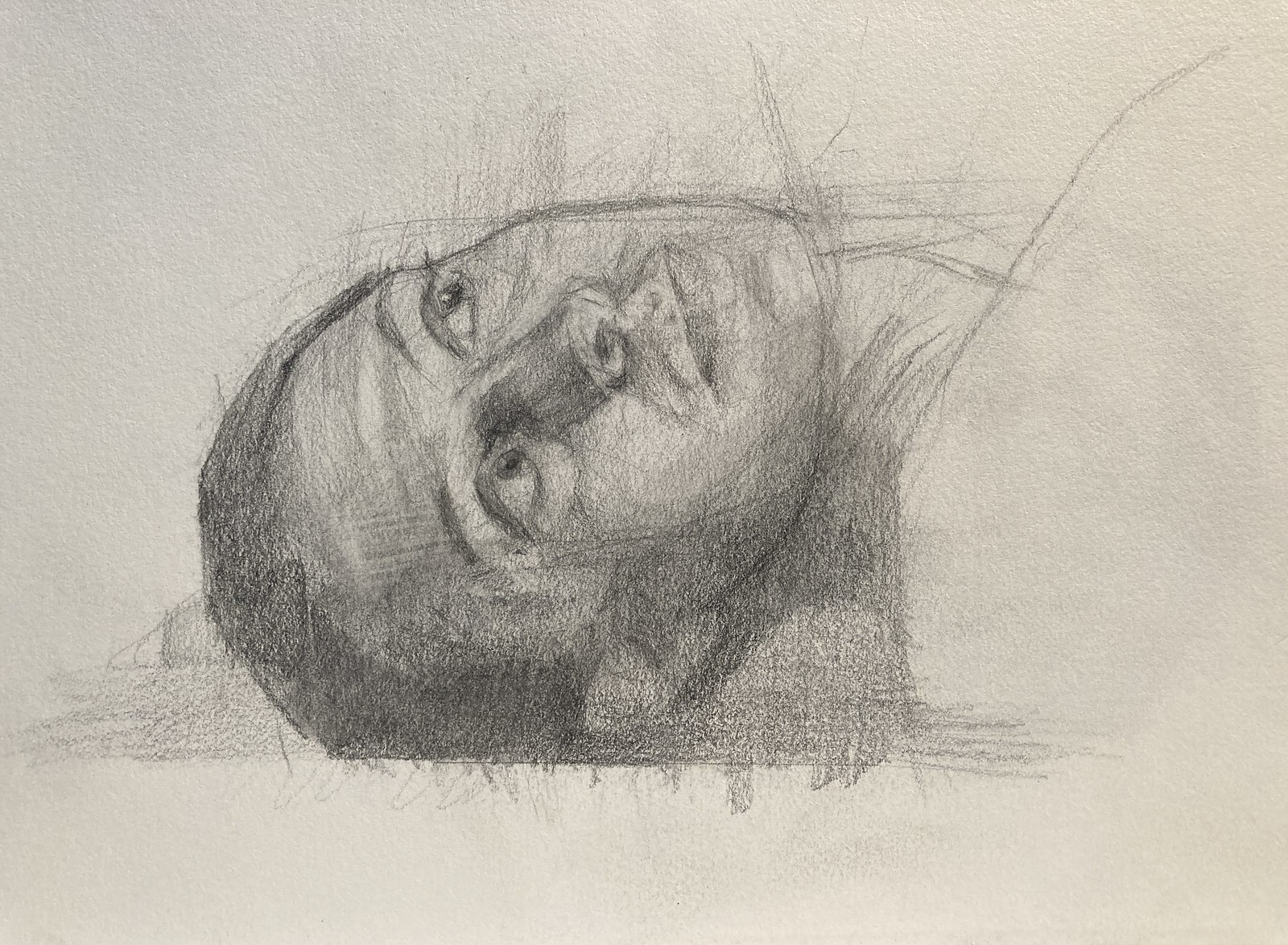The image depicts a rough pencil sketch on an off-white or gray piece of paper, likely from a sketch pad. The sketch features a person's face, who could be either male or female, with short hair and a slight grin. The individual is positioned laying down, with their head turned and eyes gazing to the left. The drawing includes darker shadows and creases, especially around the forehead and nose area, and extends to an outlined neck and shoulders, with some shadowing beneath. The overall style is loose and sketchy, with numerous scribbles and lines extending beyond the facial outline.